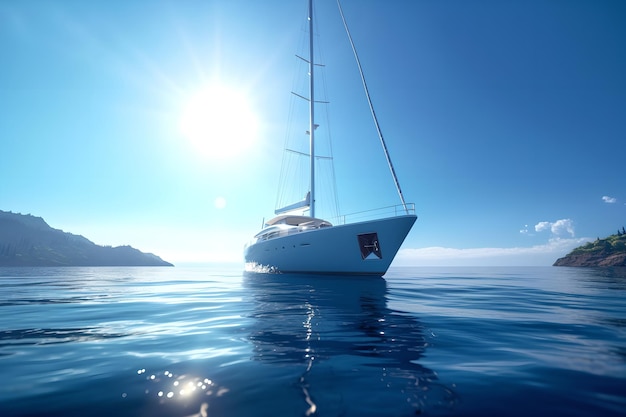A serene image showcases a white sailboat resting on calm, icy blue waters. The photograph appears to be taken from a unique perspective, possibly from another boat or even from the water itself. The sailboat is prominently centered, featuring a tall mast without any sails raised. The bow is angled slightly, pointing towards the right side of the frame, giving an almost profile view.

The sky dominates the upper two-thirds of the image, a brilliant blue expanse nearly devoid of clouds, save for some gathered at the distant horizon. Just above the horizon line, the Sun radiates bright white light, with sunbeams stretching across the sky. This sunlight also reflects crisply off the rippling water, adding a sparkling effect.

On both sides of the sailboat, gently sloping hills rise from the water's edge, with patches of green indicating tree-covered land masses. The overall scene suggests a pleasant and peaceful day, perfect for sailing, though the sailboat itself seems to be at rest, absorbing the tranquility of its surroundings.